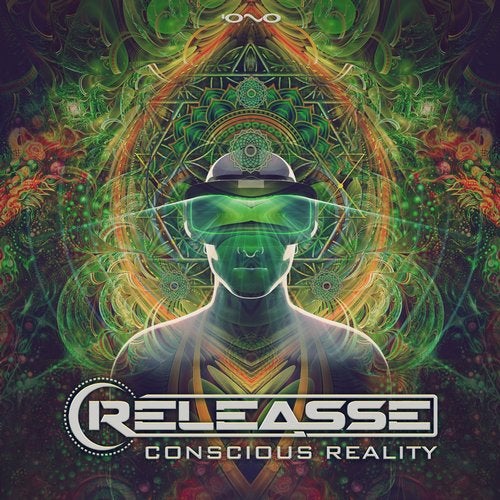This advertisement features a vividly colorful and surreal graphic, evoking the aesthetics of a video game cover. The design is predominantly green and orange with intricate swirls and patterns that resemble the view through a kaleidoscope, all set against a solid black background. Central to the image is an orange teardrop shape, outlined and adorned with varying green and orange scrolls and shapes, beginning at the top and tapering to a point at the bottom.

In the forefront stands a computer-generated, shadow-like figure of a man, donning large green goggles that emit a reflective green light. The man appears to be wearing accessories reminiscent of Egyptian jewelry in matching orange hues. The face is simple, with a straight white line representing the mouth, and the overall figure is enveloped in white outlines, cutting off at the waist. 

Conspicuously displayed across the person's chest in bold white letters is the word "R-E-L-E-A-S-S-E," which is also outlined in white. Below this, the phrase "conscious reality" is written, hinting at a connection to virtual reality equipment or an experience. The top of the teardrop-shaped background features the letters "ONO" in striking white, further adding to the enigmatic and futuristic theme of the advertisement.